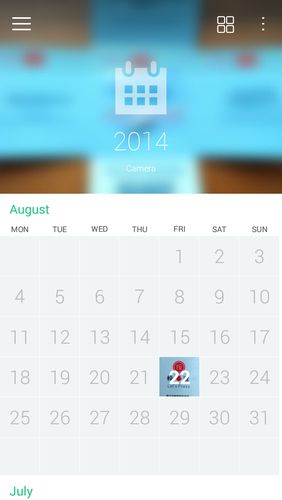The image displays a digital calendar from a website, specifically showcasing the month of August in the year 2014. The entire calendar interface is framed neatly on the screen, with the month's name "August" prominently highlighted in green text. The background features a blurry image, indistinct but providing a textured backdrop to the calendar. The date of August 22nd is clearly selected, possibly indicating an entry or a significant reminder set by the user for that day. The overall design is minimalistic, focusing on the calendar itself without any additional elements or distractions.